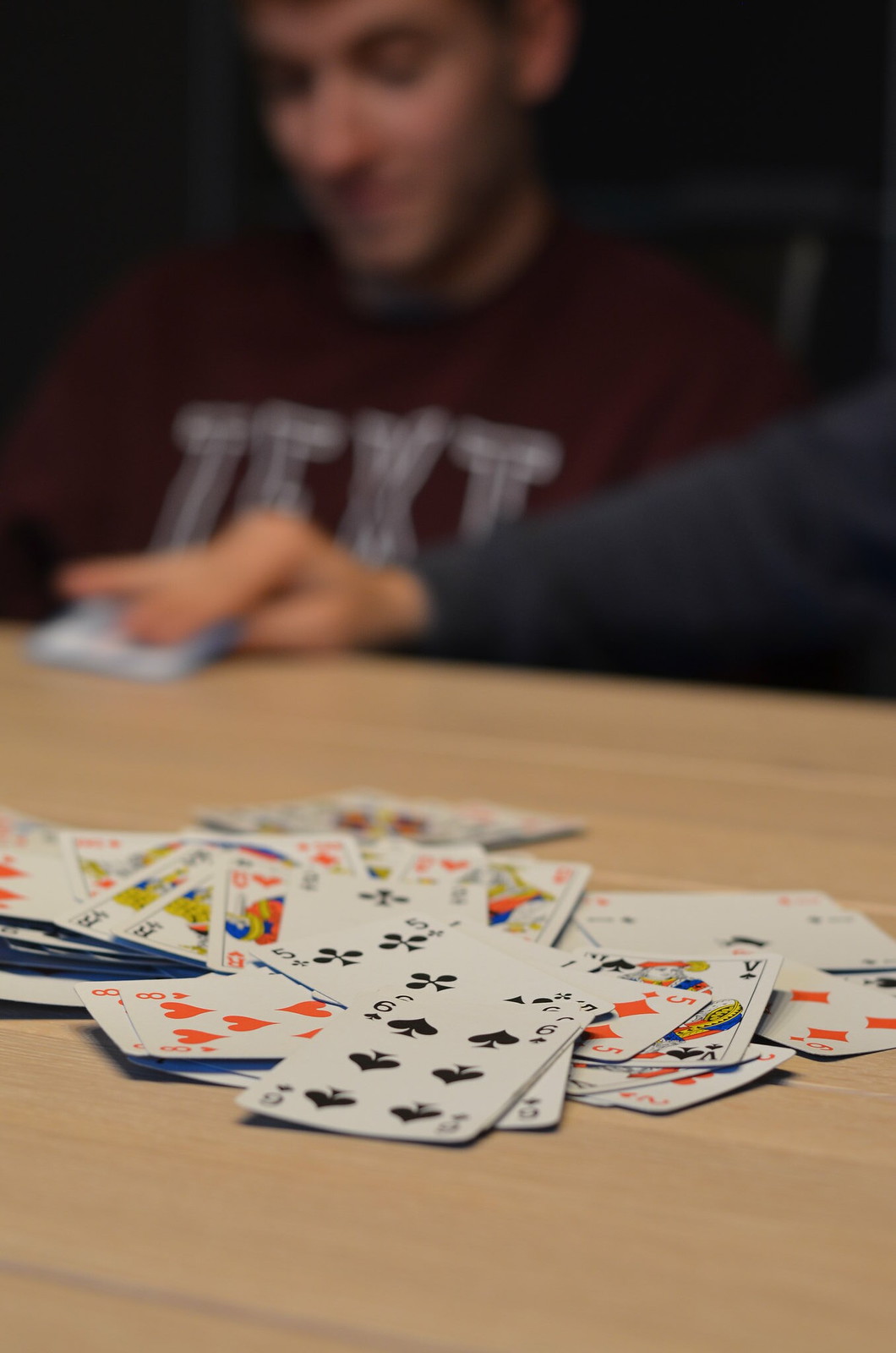This photograph, oriented vertically in a rectangular frame, is captured with a slight blur at both the top and bottom. In the foreground, a man is seated, visible from the waist up. He is dressed in a deep red sweatshirt adorned with bold, white capital letters that spell out "TEXT," though the 'E' is partially obscured by another person's hand intruding into the frame from the left. This hand, clad in a gray, long-sleeved shirt, holds a stack of bluish items.

The man in the red sweatshirt is looking down, his face absorbed in concentration, though the top of his head is cropped by the image's upper edge. The background remains dark, emphasizing the scene's intimate focus. 

In front of the man is a tan table scattered with playing cards, all face up. Centered towards the top third of the photograph, a black six of spades is prominently displayed beside a red eight of hearts. Below the six of spades lies a black five of clubs, and to its right, a red five of diamonds. The rest of the playing cards are slightly blurred, contributing to the overall dynamic yet focused composition of the image.